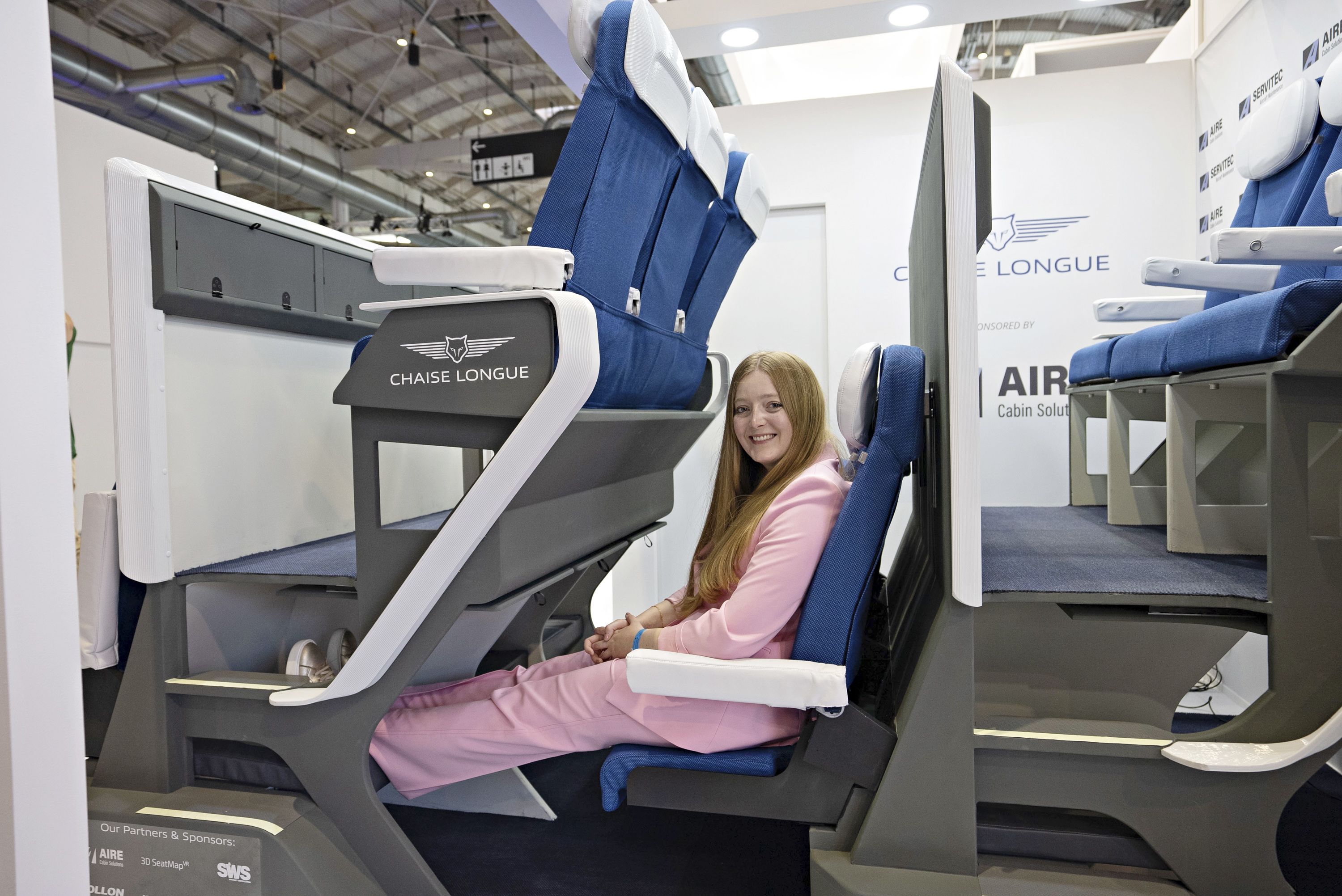The image depicts a demonstration setup showcasing a staggered seating concept, likely intended for an airline, within an airport or hangar environment rather than an actual airplane. The seating arrangement alternates in height; with each row being either raised or lowered to provide more legroom. The chairs feature blue cushions with white armrests and headrest covers. A young woman, possibly in her late teens or early 20s, is seated in a lower row, illustrating the ample legroom by fully extending her legs onto a footrest. She wears a pink pantsuit, golden shoes, and a blue armband. Her long, reddish hair is side-parted, and she is looking towards the camera with a smile. The seating area's plastic components are gray, and there is a logo displaying the phrase "chaise lounge" accompanied by an ambiguous animal face, either a fox or a cat. This photograph, taken in landscape mode, aims to demonstrate the future of airline seating comfort.